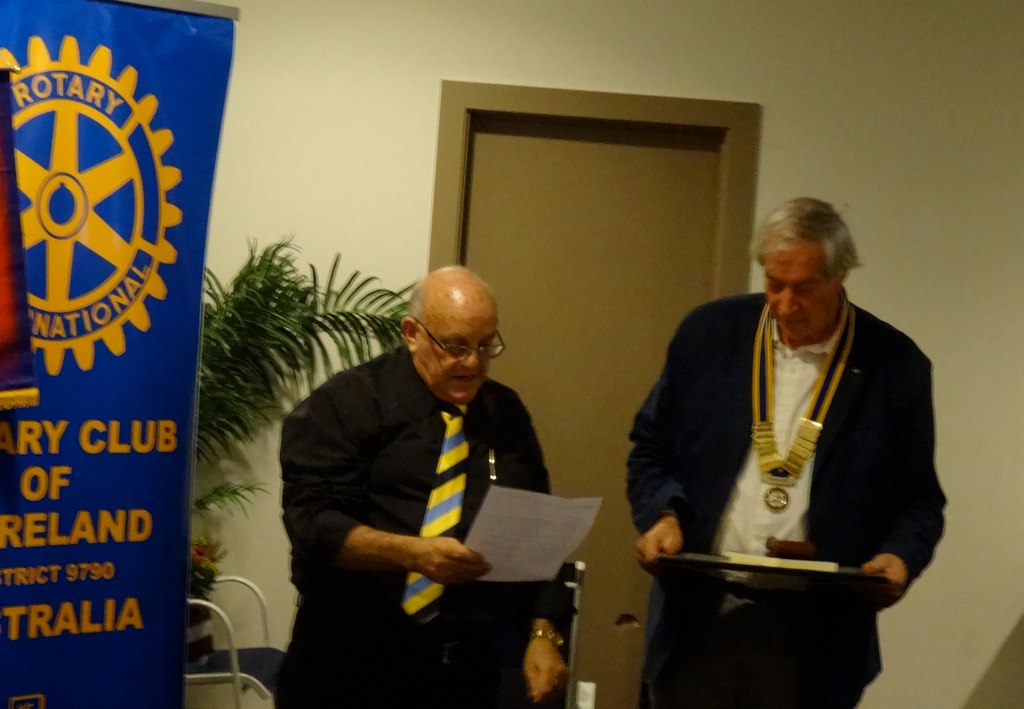In the image, two elderly Caucasian men stand at the center, both engrossed in their respective tasks. The man on the center-left is sporting a black button-up shirt paired with a yellow, blue, and black striped tie. He has a balding head with sparse gray hair, is wearing glasses, and accessorizes with a gold watch. He is reading intently from a white sheet of paper in his hands. To his right, the other gentleman, slightly taller and with short gray hair, is dressed in a white button-up shirt under a blue blazer. Around his neck hangs a blue and yellow ribbon supporting a gold circular medal positioned just below his chest. He is holding a tray with both hands, looking down at its contents, which are unclear but might resemble butter. The background features a white wall, a green plant, and a brown door to the right. To the left is a partially visible blue and yellow Rotary Club banner with a circular emblem, inscribed with "Rotary International" and likely "Rotary Club of Ireland" though partially cropped.